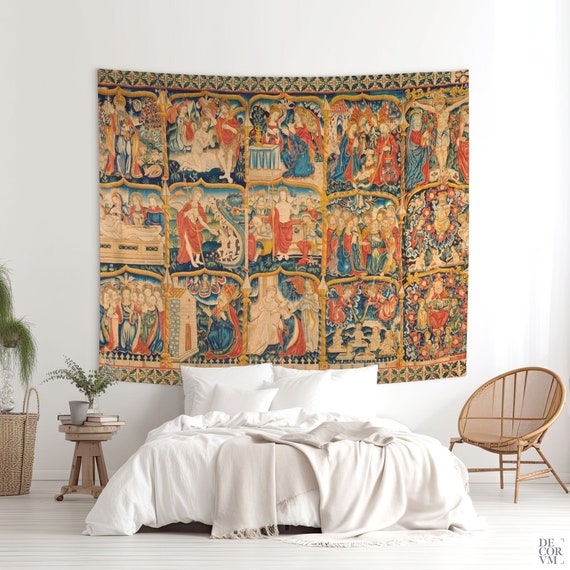This photograph captures the interior of a serene bedroom. The focal point is a low-profile bed, positioned centrally, adorned with white bedding—pillows, sheets, quilt, and throw—creating a clean and crisp aesthetic. The bed rests on whitewashed hardwood floors, their horizontal slats adding a touch of rustic charm. Looming behind the bed is a large, ornate tapestry with an indeterminate Roman style, populated by numerous figures dressed in reds, blues, greens, and cream hues, creating a historical and artistic centerpiece against the plain white wall.

To the left of the bed, a round wooden nightstand on wheels holds an artificial floral arrangement, a muted gray cup, and a few books, suggesting a cozy reading nook. Nearby, a potted fern or bush adds a touch of greenery, possibly contained in a brown wicker basket. On the right side, a wicker-style chair adds to the natural, textured elements of the room. Light seems to filter in from the right, likely through a window, adding a soft, natural illumination that enhances the tranquility. In the lower right corner of the image, the partial words "DE," "COR," and "VM" hint at a subtle decorative signature.